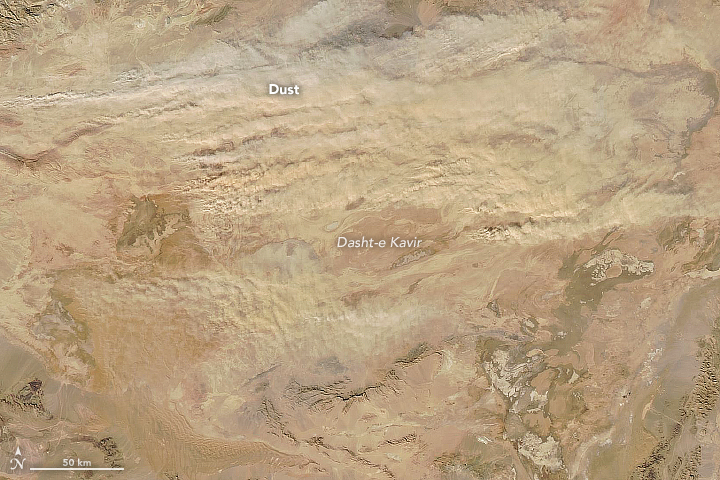The image is a highly detailed, realistic topographical map, possibly created from satellite imagery or a detailed clay model, showing various landforms in muted, earthy tones like brown, tan, beige, gray, and subtle greens. The terrain is depicted with a swirly, grainy texture, indicating the ruggedness of the landscape. In the bottom left corner, there is a scale marker showing "50 KM" next to an "N" symbol with an arrow pointing north. Centrally, the map is labeled "Dasht-e-Kavir" in white text, while the top left corner has the word "Dust." The map showcases a region resembling the Arabic desert with a mix of rocky surfaces and cracked, pocked areas that get lighter in color towards the top.